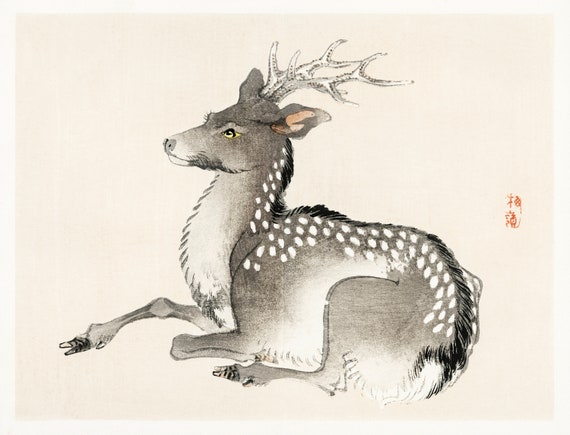This illustration features a stylized and whimsical depiction of a mature deer, rendered in a blend of East Asian ink wash painting, known as Tsutsumi-e, with colored pencil techniques. The deer is portrayed in a seated position, with its body turned to the side and its head facing forward, exuding a serene and graceful posture. Its prominent, branched antlers—consisting of seven points—emerge from between its ears, rendered in shades of white with gray and black accents to provide depth and shadow.

The deer's fur is predominantly gray with a series of distinctive white speckles running from the base of its head down its back, accentuating the form and adding texture. It has a black stripe, or mane, running from its neck to its tail, which begins bushy and black then fades into white. The legs are a darker gray with black hooves; one front leg is extended while the other is curled up, and the back leg is folded beneath its body.

The deer's facial features are highlighted by bright yellow eyes with black pupils, creating a striking contrast. Detailed fur around its muzzle is thicker and appears darker, while the ears are gray with pink interiors. The background is plain, light-colored, and potentially has a faint, pinkish hue. Japanese characters, written in red ink, are located on the right side of the image, mid-way down, likely serving as the artist's signature.

This nuanced and expressive piece merges elements of traditional East Asian artistry with detailed, three-dimensional shading, capturing both the dignity and tranquility of the majestic creature.